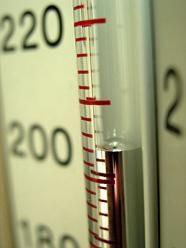The image depicts a measuring tube filled approximately halfway with a purplish liquid. Positioned vertically, the tube is transparent, likely made of glass, and features graduated markings in red. On the left side of the tube, there is a scale marked with "220," "200," and "180," with white background and black lettering. The "220" marking aligns with a prominent red line on the tube, whereas the "200" and "180" markings do not seem to match up as precisely. 

The liquid level appears to be around the 200 mark. On the right side of the tube, a single number “2” is visible, possibly indicating a different measurement system. The background on the right appears to be gray. The tube extends upwards and connects to a smaller, non-transparent gray segment, which possibly serves as a support or holder for the larger tube. 

The larger tube has intervals marked at approximately every quarter inch with longer red lines signifying significant levels, interspersed with shorter lines denoting smaller increments. As the tube narrows towards the top, it forms a slight bulb. The detailed calibration and the distinct sections of the tube suggest it is a precise scientific instrument, potentially used for measuring volumes of liquid in a laboratory setting.